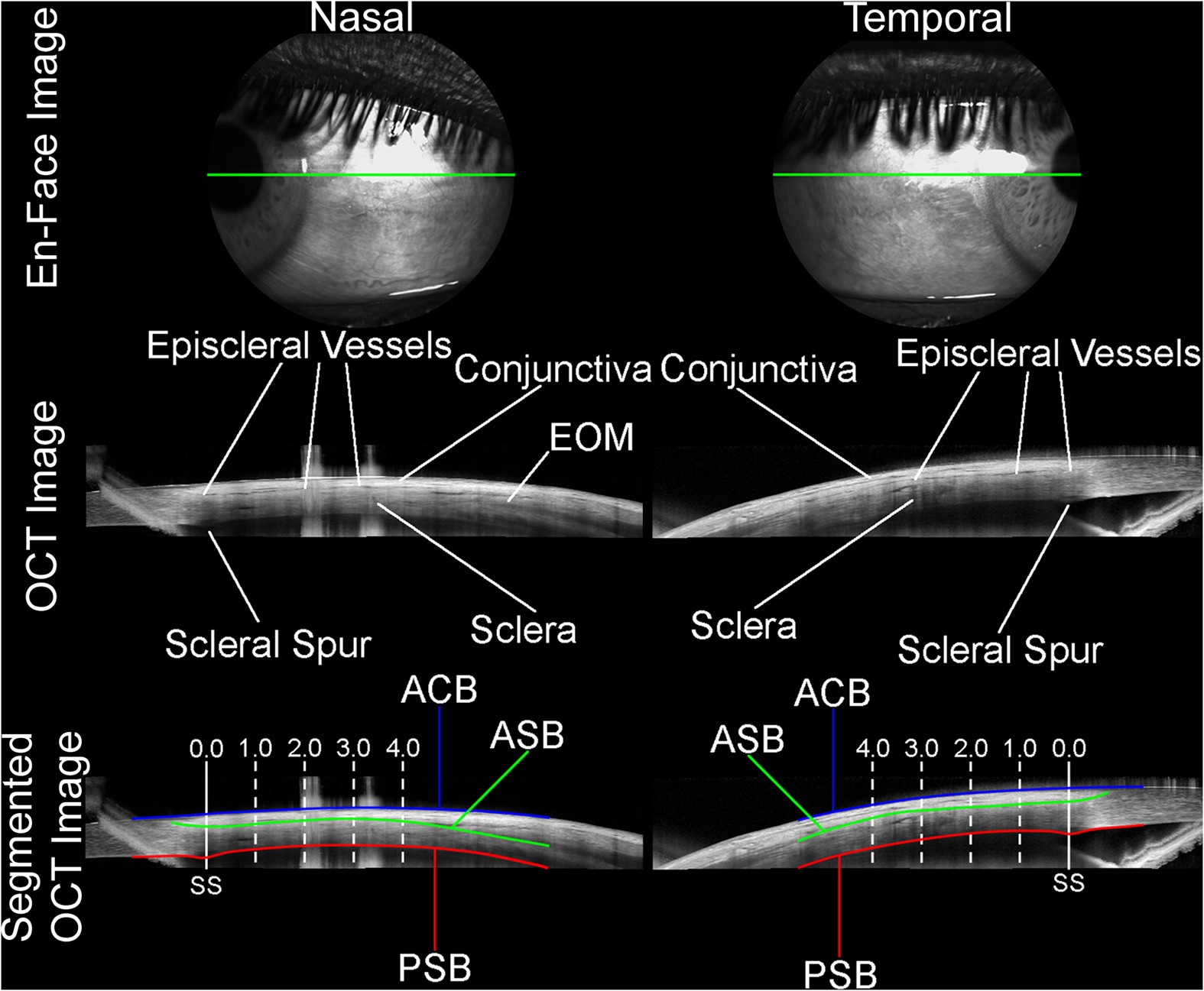Displayed against a black background, this intricate scientific diagram features two side-by-side, close-up, black-and-white images of an eyeball, meticulously labeled for medical or research purposes. The left image, labeled "nasal," shows an eyeball looking to the left, while the right image, labeled "temporal," shows an eyeball looking to the right. Each eye is bisected by a bright green line running horizontally through the center. 

Below each eyeball, text points to rod-like structures representing different parts of the eye, and beneath these are various labeled lines in red, green, blue, and white (some dotted). These lines and labels map out specific anatomical features such as episcleral vessels, conjunctiva, EOM (extraocular muscles), scleral spur, and sclera, indicating the complex internal structures of the eye. 

On the right side of the overall image, text aligns vertically from bottom to top, reading "segmented OCT image," "OCT image," and "end face image," correlating with different sections of the detailed ocular analysis. The entire diagram appears well-suited for detailed medical or scientific examination of ocular anatomy.